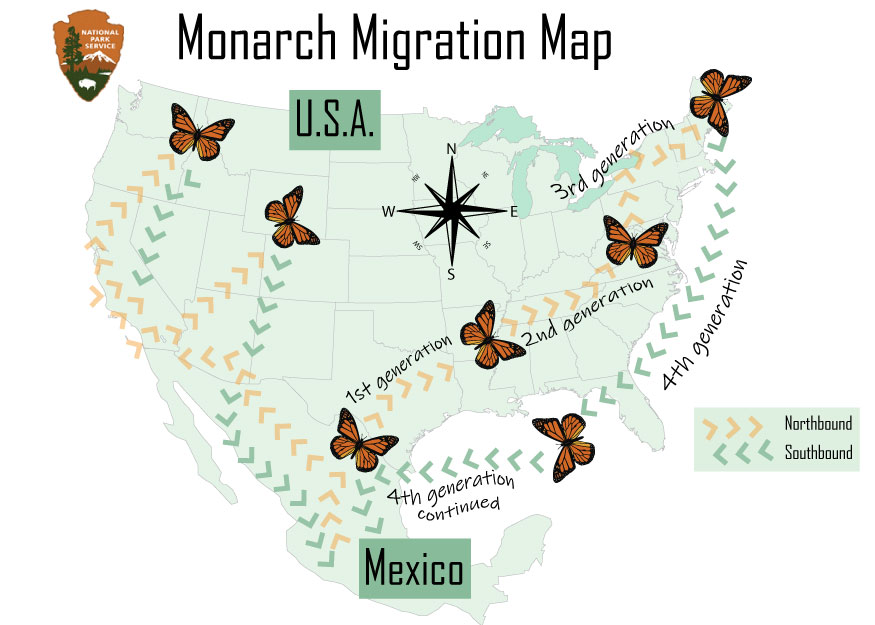This detailed illustration depicts a monarch butterfly migration map covering the United States and Mexico, produced by the National Park Service, as indicated by their arrowhead logo in the upper left corner. The map prominently features the title "Monarch Migration Map" in black text at the top. The map itself is rendered in a grayish-green color and includes border lines separating different states. Text boxes label "USA" above the United States and "Mexico" above Mexico.

Six black and orange monarch butterflies are illustrated along their migratory path. Starting in the Texas-Mexico border region, the journey is marked by generational stages. The first generation moves north from Texas. The second generation continues eastward, passing through Tennessee and Virginia. The third generation heads further northeast, reaching as far as Pennsylvania and Maine. The fourth generation loops southward over the ocean, passing through Florida and the Gulf, while the fourth generation continues back towards Mexico along the western seaboard of the United States.

An additional key on the map uses orange arrows to indicate northbound movement and green arrows for southbound migration.